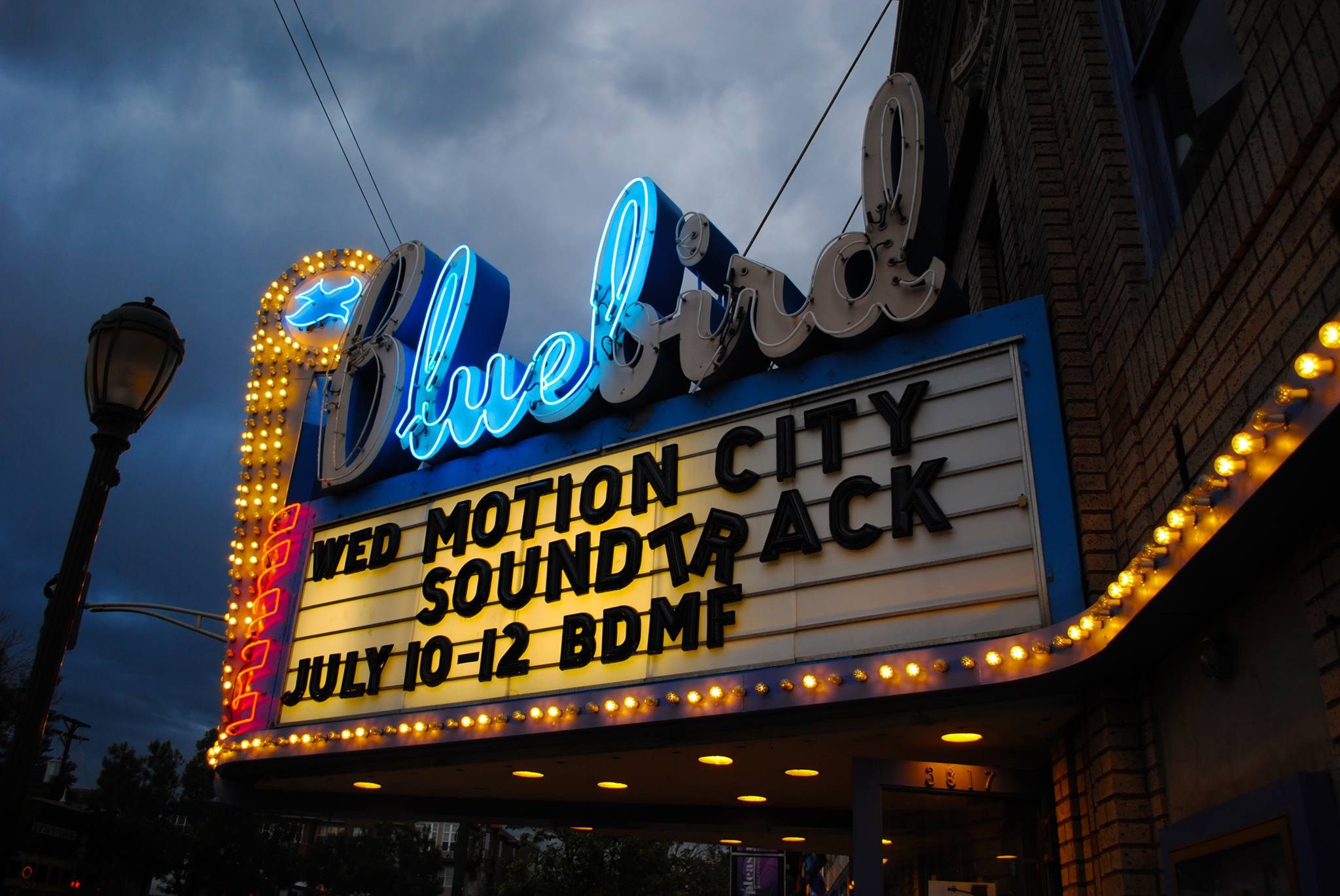The image features a marquee for the Bluebird Theater, captured in a close-up shot at nighttime under a dark, cloudy sky. The theater's name, 'Bluebird,' is displayed in neon lights, though many of the tubes are burnt out, leaving only the letters 'L-U-E' and part of the 'B' visible. Despite the missing illuminations, the full name is discernible. Adjacent to the text is a vertical design featuring a bluebird atop an elevated area. The marquee advertises an event: 'Wednesday: Motion City Soundtrack, July 10th-12th, BDMF.' Some of the letters are slightly askew, creating an uneven appearance.

The structure of the marquee includes an overhang ceiling embedded with approximately 10-12 lights. Surrounding the marquee's base and sides are additional lights, some of which flash intermittently and others are not fully lit, suggesting that the sign could benefit from repairs. The theater building itself is made of brick, and a nearby street lamp, positioned to the left of the sign, remains unlit. The ambiance suggests a slightly neglected yet iconic venue, with the potential for lively events despite its weathered appearance.